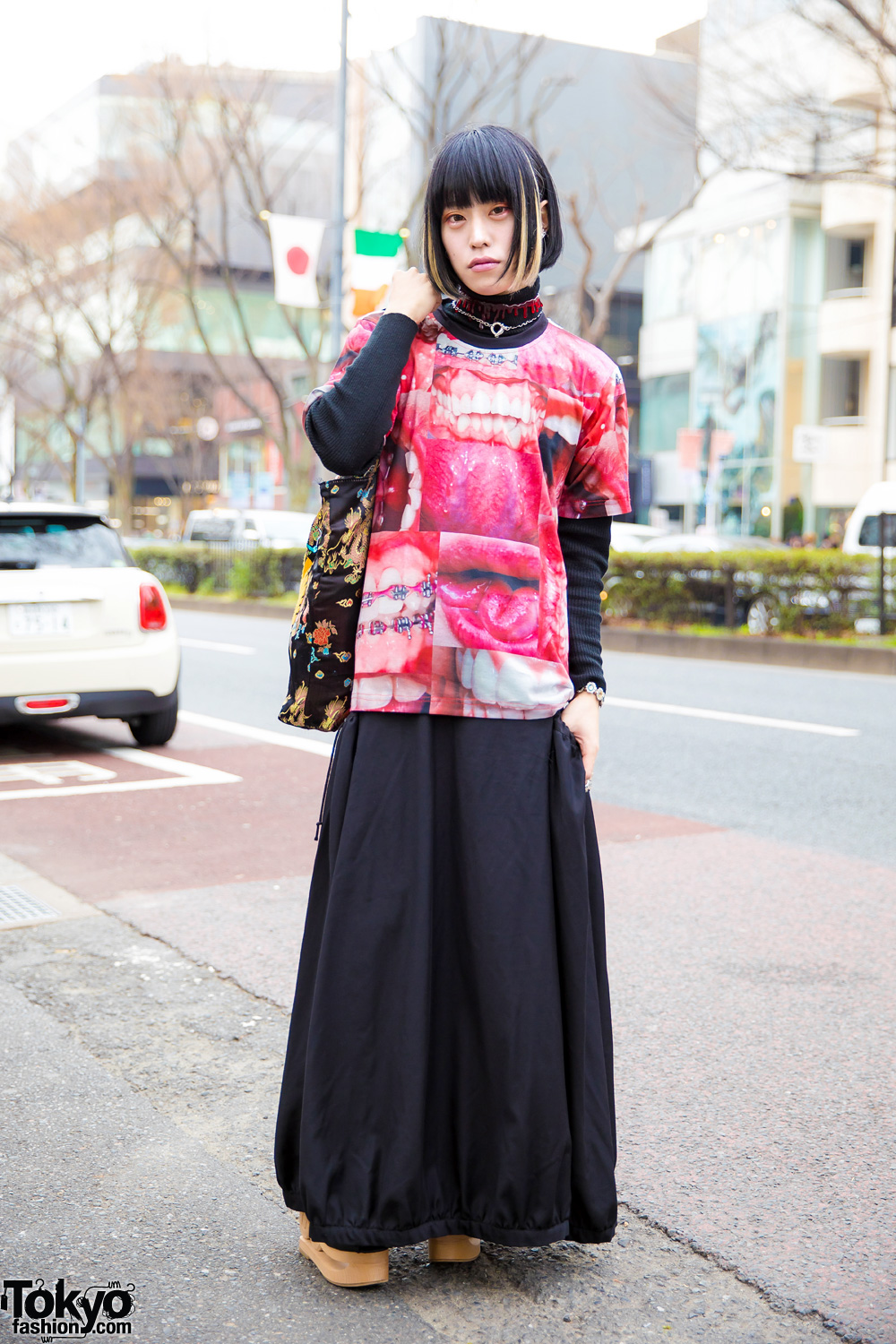In this visually arresting photo set against a muted cityscape backdrop in Japan, a woman stands confidently on a sidewalk, looking directly at the camera with a neutral expression. She sports a chin-length blunt black bob with straight bangs and distinctive  blonde highlights framing her face. Her outfit is a striking mix of styles and colors: she wears a long black skirt paired with a long-sleeved black dress, over which she dons a vibrant pink-red tie-dye-patterned short-sleeve t-shirt adorned with an unusual and eye-catching design resembling the inside of human mouths, complete with gums and teeth. Around her neck is a silver choker necklace featuring a small charm, possibly a heart. She completes her eclectic look with a pair of brown Timberlands boots and carries a black tote bag decorated with a floral print in yellows and oranges, emblazoned with the text "TokyoFashion.com" at the bottom. The scene captures various elements of urban life, including buildings in the distance, the back of a white car parked on the road, and flags of Japan and Ireland visible against the muted skyline.